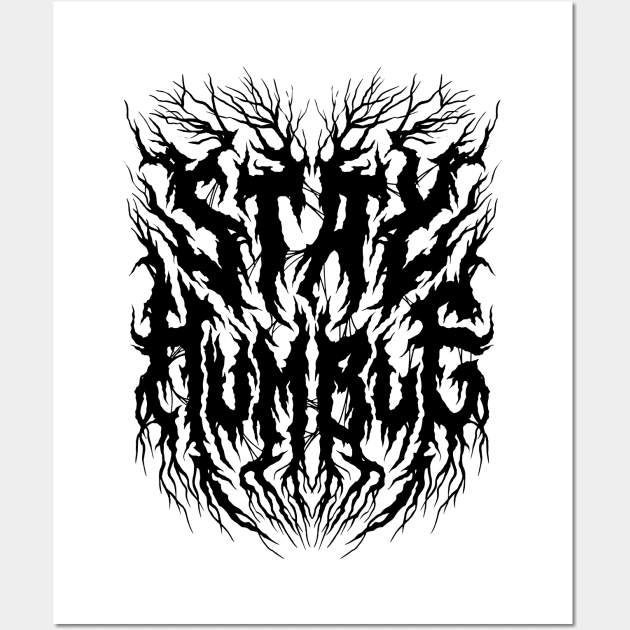In this detailed black-and-white illustration, a piece of white paper rests on a light gray platform. The artwork features an abstract, intricate design of black tree limbs forming the words "STAY HUMBLE." The tree limbs interweave to create a shield-like shape that flares at the top, concaves on the sides, and tapers at the bottom. These scraggly, pointed branches vary in thickness and orientation, some even growing off other limbs, lending a dynamic and textured appearance to the typography. The word "STAY" is positioned at the top of the picture, while "HUMBLE" sits below it. The black tree limbs and branches create an eye-catching contrast against the white background, making the letters STAY HUMBLE appear pronounced yet integrated into the organic form of the artwork. The overall style reflects a blend of graphic design and typography, creating a visually compelling piece that emphasizes the message in a unique and artistic manner.